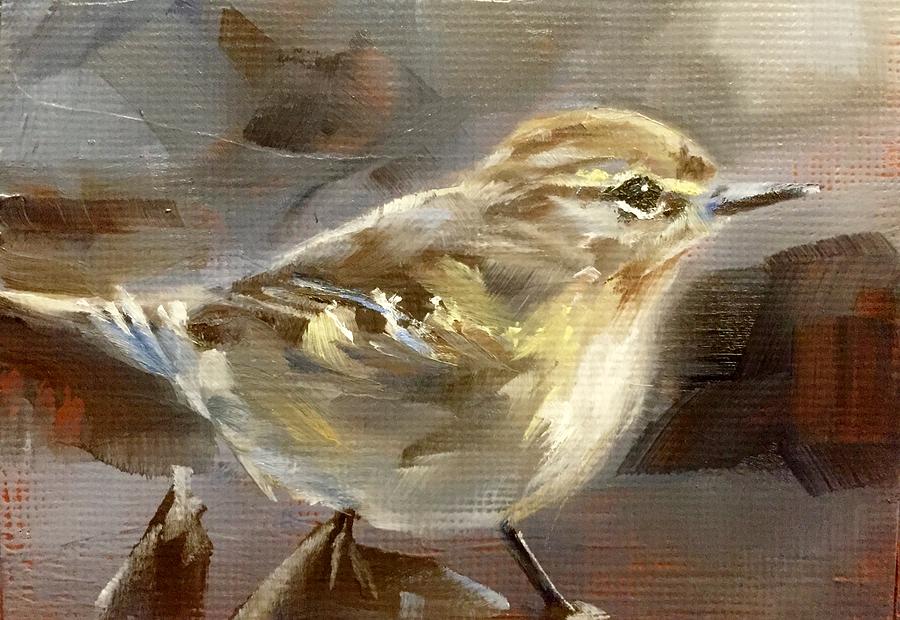This image is a close-up of a square painting, without a border, depicting a small bird in profile facing right. The bird's upper body is predominantly brown with a textured brown and yellow wing, while its belly is white. It has a black eye highlighted by a slender horizontal yellow line and a narrow pointed black bill. The legs and feet are also black. The background is abstract, a blend of brown, blue, and gray smudges with no definitive form. The canvas's woven texture is visible through the paint, creating a grid-like, matte appearance across the entire image, emphasizing the depth and texture of the painting.